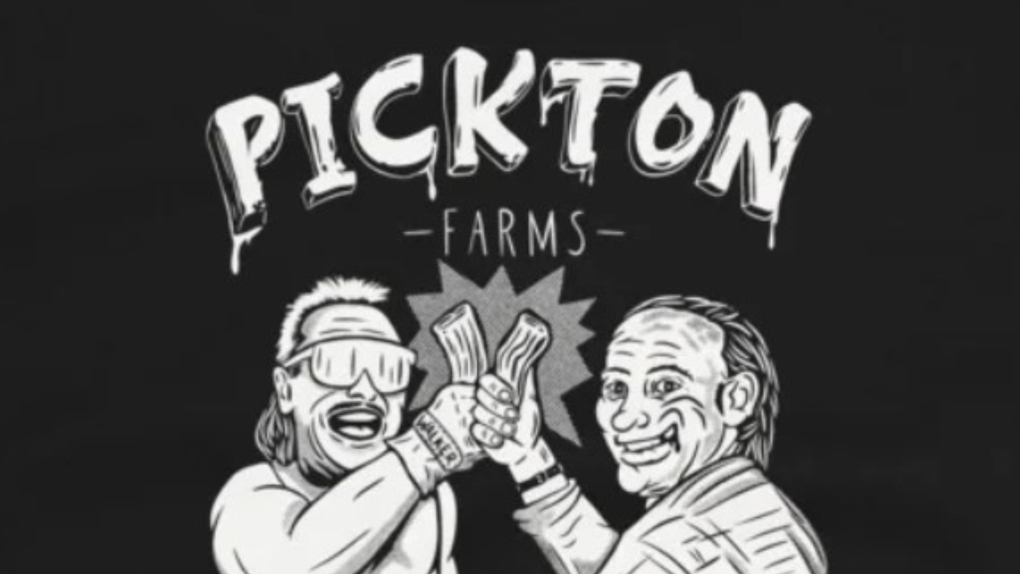The black and white drawing in this poster showcases an advertisement for "Picton Farms," with the name prominently displayed at the top in large white letters, "Picton," followed by "Farms" in smaller text. The design has a cartoonish and somewhat sketch-like aesthetic, with noticeable details like what appears to be spit dripping from some of the letters. Set against a black background, the image features two men at the bottom. The man on the left sports spiked hair, shiny sunglasses, gloves with indistinguishable text, and possibly a tank top, grinning widely while holding what could be a stick or jerky. The man on the right, older and also smiling broadly, is dressed in a jacket and a watch. Both men are depicted as if they are fist bumping with the food items in their hands, possibly indicating a celebratory or triumphant moment. The overall image is rendered in shades of black, white, and grey.